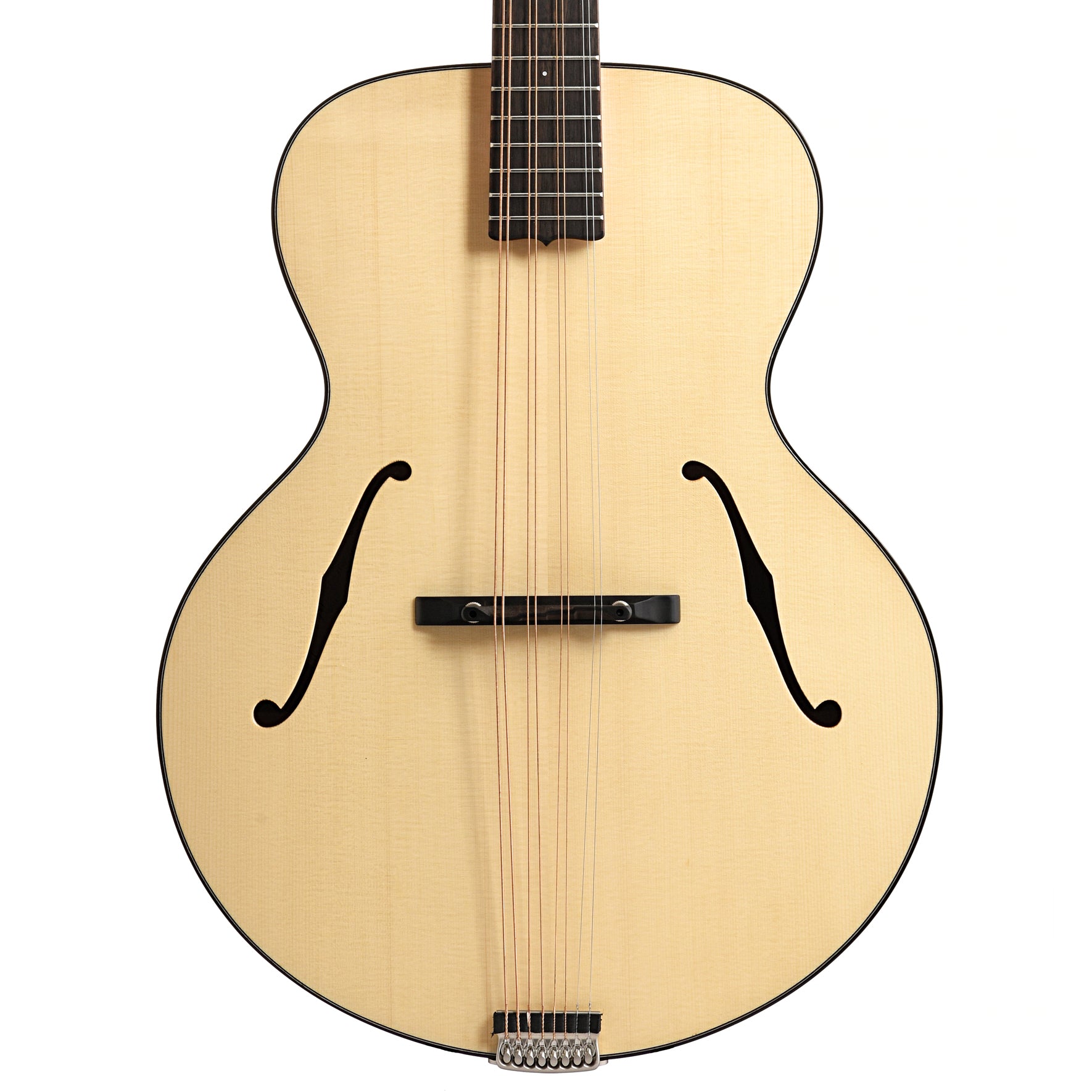The image depicts the body of an unusual guitar with eight strings, arranged with two bass strings, two high-tone strings at the bottom, and four strings in dual pairs in the middle. The guitar's body is tan, possibly made of birch wood, though the exact material is unclear. The bridge, fastened securely, is also wooden. The instrument features a distinctive black spiral design on both sides and clef note-shaped sound holes. The neck and tuning pegs are not visible, emphasizing the unique aspects of the body itself, which somewhat resembles an oversized ukulele.